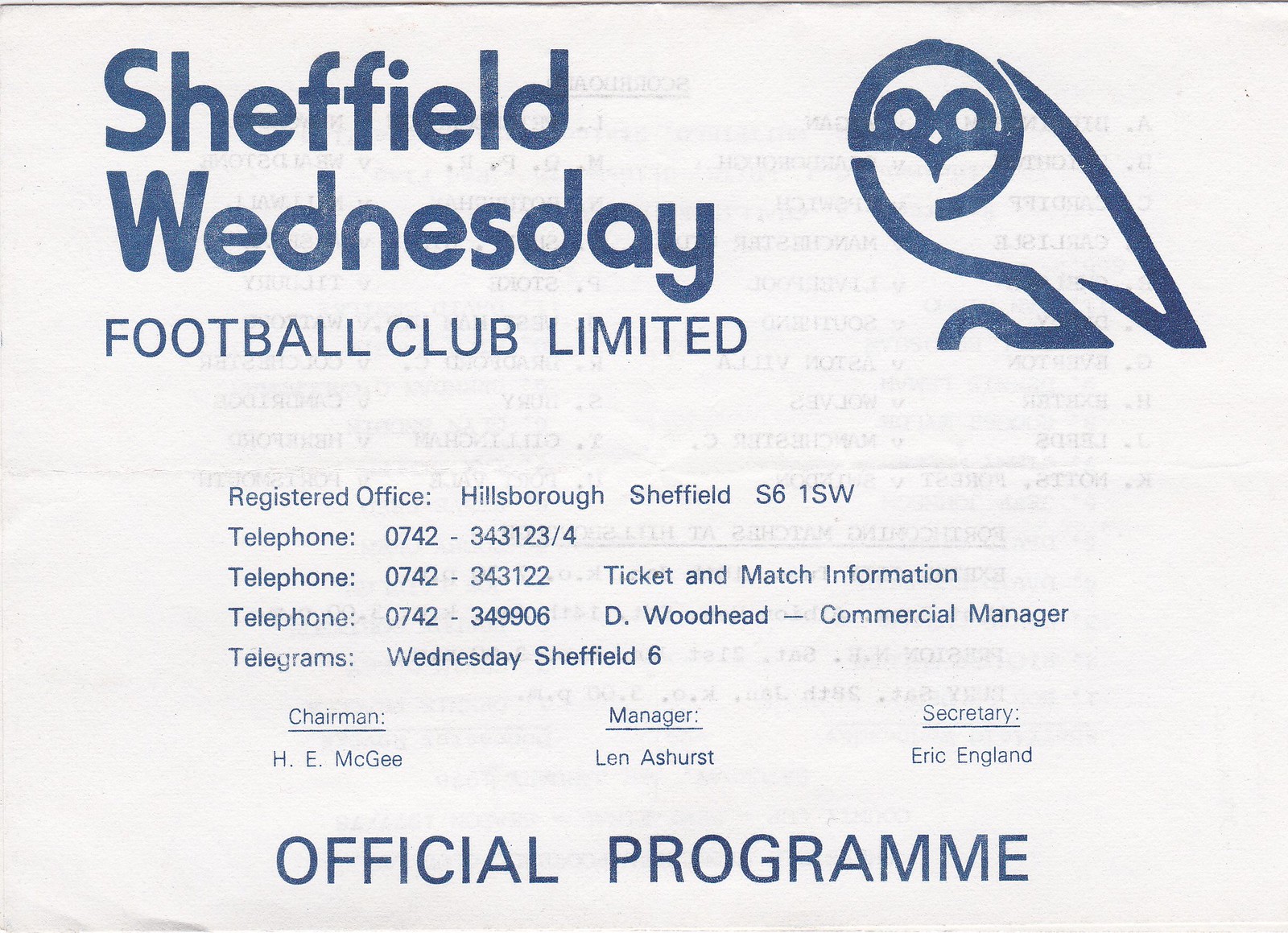The image is an official program cover for Sheffield Wednesday Football Club Limited, a soccer team based in England. The design is quite simple, featuring blue ink printed on a white piece of paper. Dominating the upper left section in large blue text is the name "Sheffield Wednesday," followed by "Football Club Limited" in smaller print. The top right corner showcases a stylized logo of an owl, facing forward, symbolizing the club's mascot.

Below the main header, the club's registered office address is listed as "Hillsboro, Sheffield, S6 1SW," along with multiple telephone numbers for different inquiries, including general information and ticketing (0742-343123, 0742-343122, 0742-349906). The telegram contact is provided as "Wednesday Sheffield 6."

Key personnel are mentioned, including the Chairman H.E. McGee, Manager Len Ashurst, and Secretary Eric England. The layout concludes at the bottom with "Official Programme" spelled with two 'M's, prominently displayed in bold blue text, emphasizing the official nature of the document.